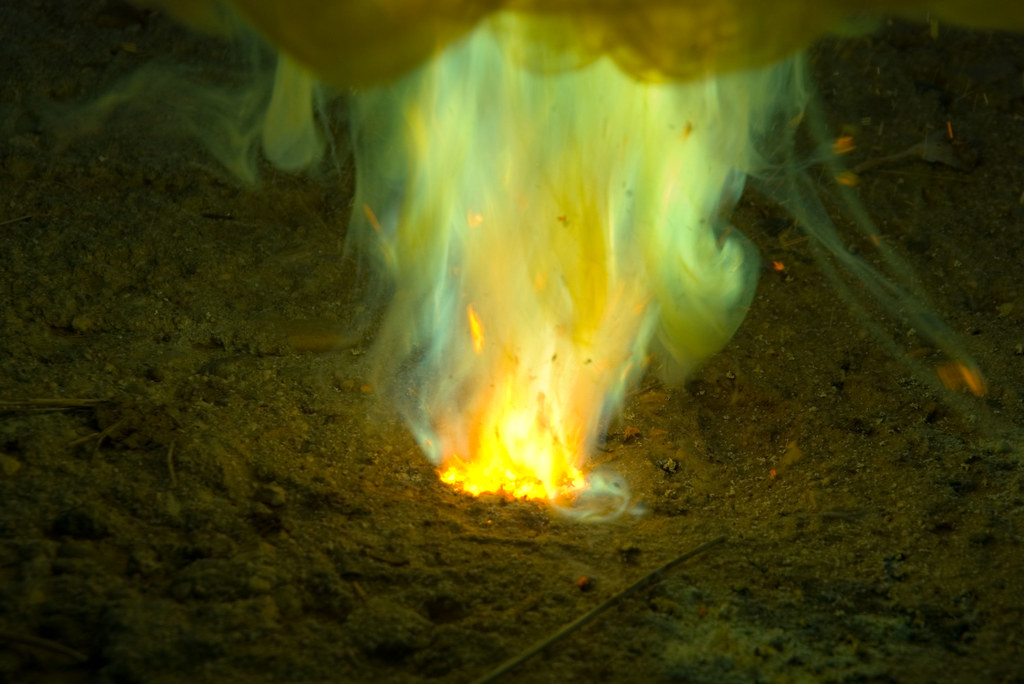Against the backdrop of a moonless night, this photograph captures a small, contained fire set on a darkened beach. The sand and gravel, barely visible in the low light, frame the vivid spectacle of the flame. At the base, the fire burns a deep orange, casting an eerie glow that illuminates the surrounding area. The upper part of the flame transitions into a neon green hue, which, combined with the mustard-yellow smoke swirling around it, creates an otherworldly atmosphere. There are no discernible sources of fuel, like firewood, making the fire's origin somewhat mysterious. The thick smoke, colored by the strange green and yellow hues, rises vertically against the pitch-black background. Scattered on the ground are sticks from fallen branches, adding to the scene's natural yet oddly surreal quality. No one appears to be present to tend the fire, enhancing its enigmatic and slightly eerie ambiance.